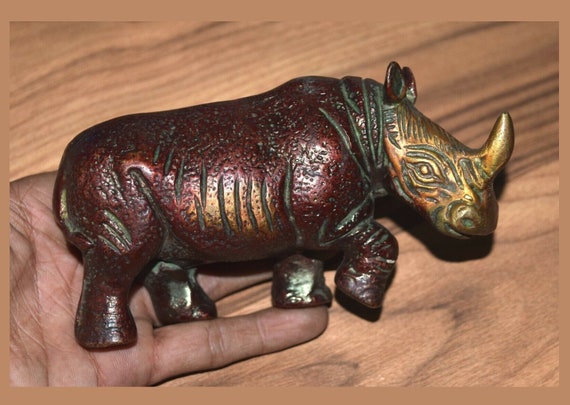This photograph captures a detailed sculpture of a rhinoceros, clasped in an open palm with only the pinky finger visible. The statue, which appears to be made of bronze, boasts an intricate design. The head of the rhinoceros transitions from a vibrant yellow to an orange hue, complete with a horn and meticulously etched features, including the mouth, nose, eyes, and ears. Moving towards the body, the colors shift to a rich mix of burgundy and yellow, accented with green stripes and hints of bronze around the stomach area. The front left foot is lifted as if the rhinoceros is in mid-stride, while the other three feet are grounded. The backdrop features a wooden tabletop with prominent dark grain patterns, enhancing the overall composition of the image.